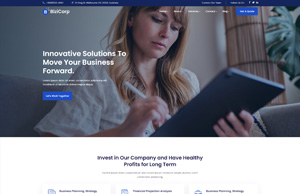This is a small screenshot of a website displaying a professional layout. At the top, there is a blue navigation bar featuring a few unreadable text options and a circular blue logo with the word "Core" next to it. To the right of the navigation bar, there are five white menu options followed by a blue button with white text.

Below the navigation bar, there is a large hero image of a woman in her early 40s with long, dirty blonde hair, sitting on a couch with a plant beside her. She is wearing a white top and holding a pen while looking at a tablet. The image is accompanied by a headline that reads, "Innovative solutions to move your business forward," and a subline text beneath it. Below the subline, there is a blue call-to-action button.

Following the hero image, a text section says, "Invest in our company and have healthy profits for the long-term," in small, centered text. Below this text, three callout options are displayed, though their details are unreadable. Despite the screenshot being very small, approximately two-and-a-half inches wide on the monitor, a surprising amount of detail can be discerned.